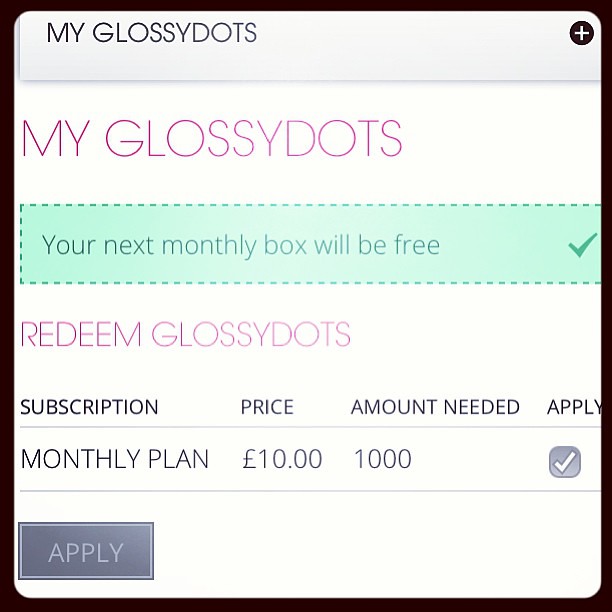The image is a screen grab, likely from a website or a mobile app, displaying a white background bordered by a black frame. At the top, "My Glossy Dots" is written in black text. Below that, "My Glossy Dots" appears again in a larger, purple font. A green banner follows, containing the text "Your next monthly box will be free" in darker green and accompanied by a green check mark. Further down, in purple, it reads "Redeem Glossy Dots." Beneath that, a series of words in black text— "Subscription," "Price," "Amount Needed," and "Apply" —are listed from left to right. Below this, "Monthly Plan £10" and "Amount Needed £1,000" are shown in black text, next to a small gray check mark. In the bottom left corner, there is a small, gray rectangle with lighter gray text that says "Apply." The entire layout is surrounded by a dark brown border that contains seven horizontal lines, dividing the sections.